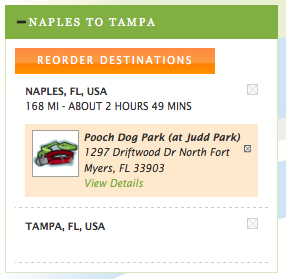The image displays a detailed itinerary for a trip from Naples to Tampa. At the top, there is a green banner with "Naples to Tampa" written in white font. Below the banner, the background is white. 

Underneath, there is an option labeled "Reorder Destinations" in white text on an orange background. Following this is the trip's starting point, "Naples, Florida, USA," noted in black text, along with the distance of "168 miles" and the estimated travel time "about two hours and 49 minutes." To the right of this information is a small square with an X inside.

Further down, a light tan rectangle contains detailed information about a waypoint: "Pooch Dog Park at Judd Park," located at "1297 Driftwood Drive, North Fort Myers, Florida, 33903." The phrase "View Details" is written in green, and there is another small gray box with an X to the right of this information. Additionally, an icon is present next to the Pooch Dog Park details; it appears to be a small graphic, possibly a red dog collar, along with other green and gray elements, all placed within a white square overlapped by a gray rectangle on the light tan background.

Below the tan rectangle, a gray dotted line segments the itinerary. The next destination, "Tampa, Florida, USA," is listed in black text. To the right of this, there is another small gray box with an X. The section concludes with another gray dotted line running underneath it.